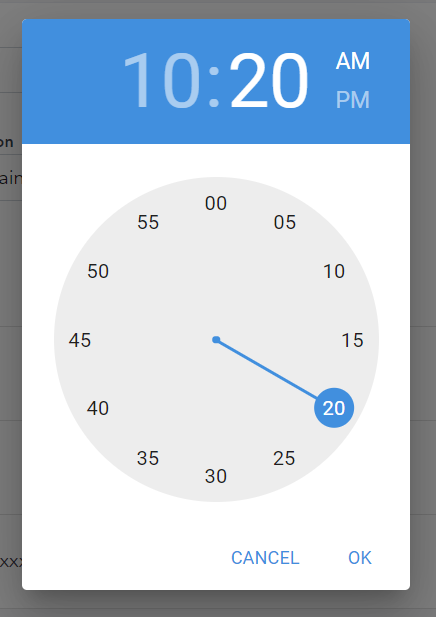A digital clock interface is displayed on a device screen. At the top of the screen, the time reads 10:20 AM, with "10" and the colon colored in light blue, and "20" in white. The "AM" indicator is illuminated in white while the "PM" indicator, which is not active, appears in light blue. The time display is set within a light bluish rectangular background.

Below the rectangular time display, a large gray circle fills the center of the screen, functioning as a minute selector. Marked around the perimeter of the circle in 5-minute intervals, starting from the top, the numerals "00," "05," "10," "15," "20," and continuing around to "55" denote the minutes. The numeral "20" is highlighted with a blue circle to indicate the current minute setting of 10:20 AM.

Additional control buttons, "Cancel" and "OK," are located at the bottom of the interface, both rendered in blue. The overall design of the digital clock interface utilizes a cohesive color scheme of light blue and white for clarity and ease of use.